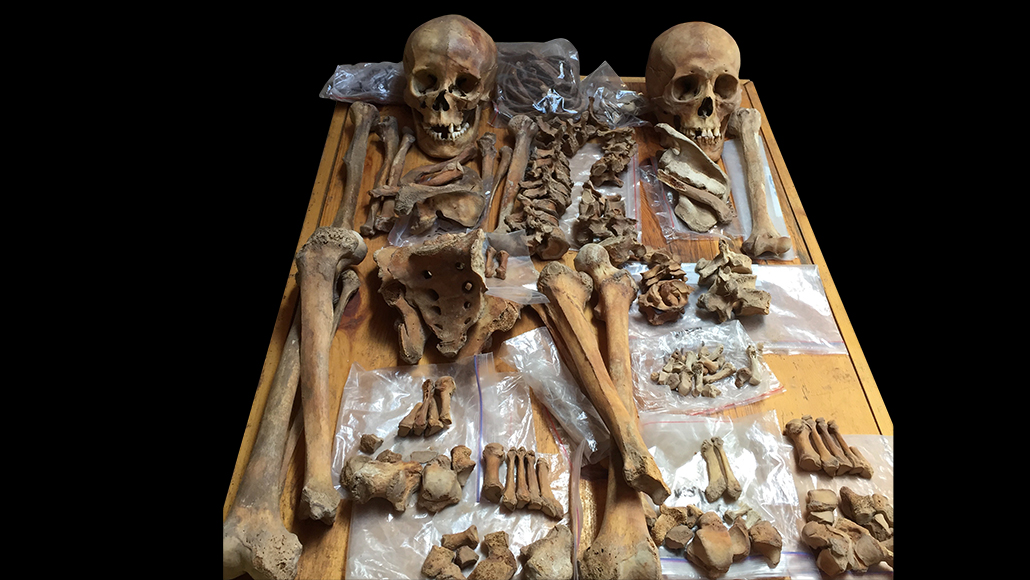The photograph showcases two human skeletons meticulously laid out on a brown wooden table against a stark black background, creating a high-contrast effect. Both skeletons are spread out side by side, their bones sorted and grouped by size and anatomical location. The presence of two skulls confirms that these are indeed two separate sets of remains, with one being more complete than the other. The bones, displaying a faded brownish-ivory hue, are accompanied by clear plastic Ziploc bags underneath and around them, containing smaller fragments. The skull on the left is missing most of its top teeth and a bottom tooth, while the skull on the right is only missing one top tooth. Despite the missing pieces, especially noticeable on the right-hand side, the main structures mostly retain their anatomical order, with the larger bones like those of the arms and legs grouped together, though the ribcages are disassembled. The layout and careful grouping provide a detailed and organized view of the skeletal remains.